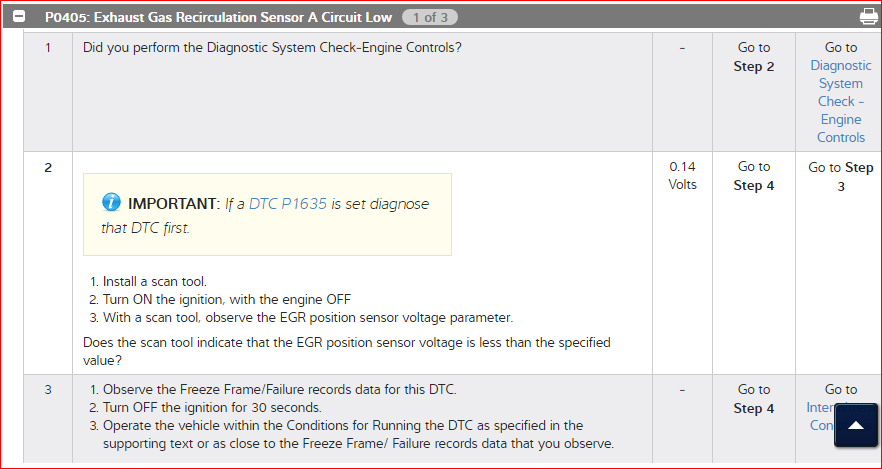The screenshot depicts a diagnostic interface on a computer screen, bordered by a thin red line forming a rectangular perimeter. A gray border across the top houses a minus icon on the far left, accompanied by the text "PO 405 Exhaust Gas Recirculation Sensor A Circuit Low," followed by "1 of 3" in a light gray circle. On the far right of this border, there is a small white printer icon.

Below this header, the main part of the screen is divided into three horizontal sections. The first and third sections are gray-shaded, while the middle section is white. Each section is further divided into five columns. The left-most column in each section lists numerical steps: "1, 2, 3." The next columns provide detailed diagnostic information and system checks.

Within the middle sections, various steps are listed, such as "go to step 4" and "go to step 2," guiding the user through a diagnostic process. The right-most small columns include additional details related to these steps.

Centrally positioned in the middle section is a yellow block labeled "Important," with a blue circle next to it, containing critical information highlighted for emphasis. Additionally, there is relevant textual data presented either for personal reference or printing.